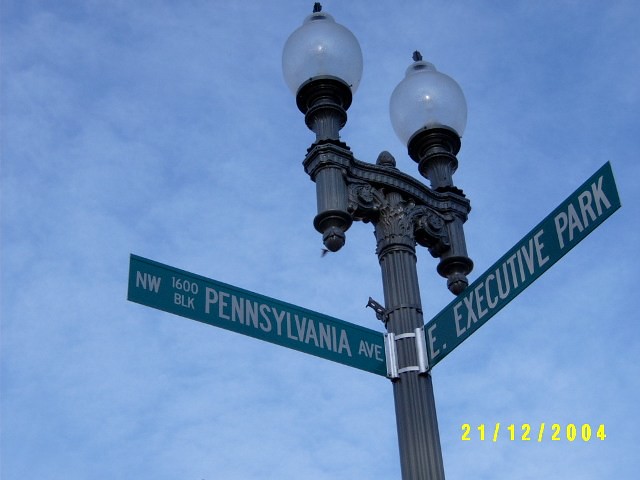This photograph, likely taken in Washington, D.C., captures a striking view looking upwards at an ornate street sign post against a predominantly blue sky with scattered white clouds. The post is crafted from what appears to be bronze or brass, adorned with intricate carvings and decorations. At the top of the post, there are two extensions, each topped with an elegant, glass-encased light bulb. The street sign on the left reads "Northwest 1600 Block Pennsylvania Avenue" in white letters on a green background, while the one on the right reads "East Executive Park" in a similar design. The overall composition highlights the elaborate design of the street post and the serene sky in the background.